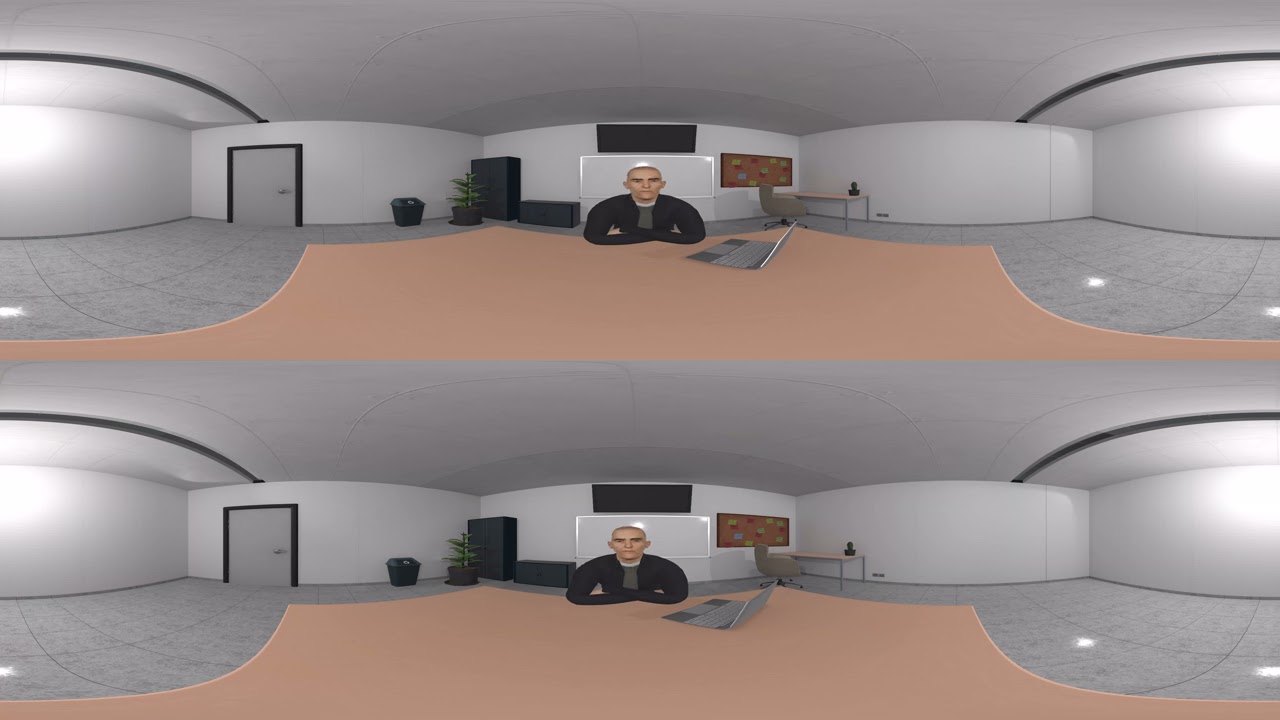The image is a detailed, computer-generated or cartoonish graphic, split horizontally and duplicated, creating an identical upper and lower half. It depicts a spacious office with white walls, a white tiled ceiling, and a grey tiled floor. In the central part of the image, a bald Caucasian man with a stern expression sits at a beige desk. He wears a dark jacket over a differently-colored shirt (described variably as green and black). The man has short hair and is leaning slightly forward with his arms crossed, positioned in front of a silver laptop.

Behind the man, there's a whiteboard on the wall with a TV screen mounted above it. To his left (viewer’s right), there is a corner with blue shelving, a plant (possibly artificial), and a garbage can. To the man’s right (viewer’s left), there is a small empty table and a beige chair, as well as a bulletin board with various post-it notes. In one corner of the room, there’s a grey doorway with a black trim, and at the very far edges of the image, lights are visible on the side walls. The lower half of the image is a repeat of the upper half, with a slight variation in the man’s head tilt, highlighting the duplicative nature of the scene.